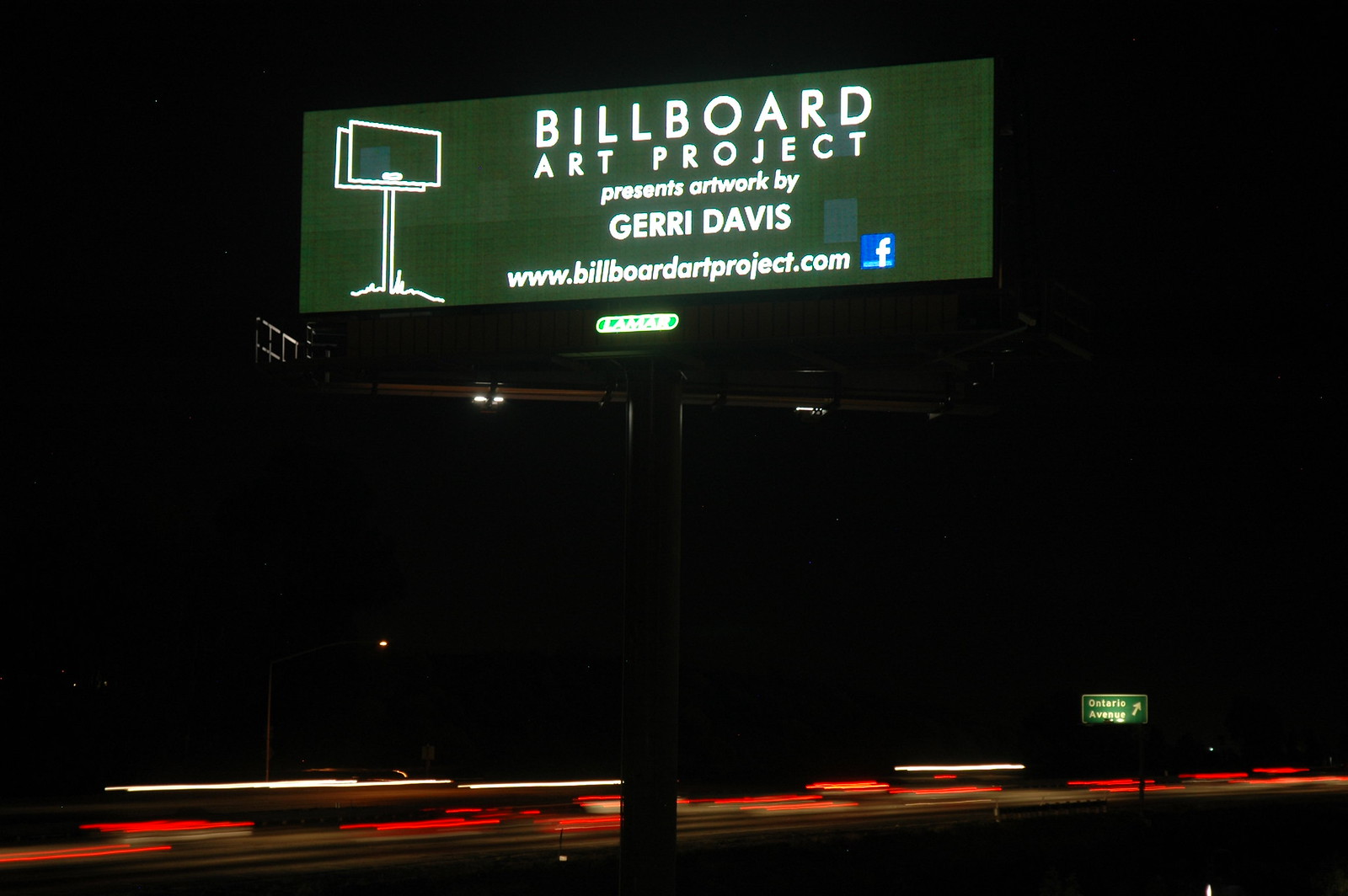This night-time photograph captures a green billboard illuminated against a pitch-black sky, featuring the text "Billboard Art Project presents artwork by Jerry Davis," alongside the website "www.billboardartproject.com" and a Facebook logo. The billboard also displays a white illustration of a billboard on a post, with some grass depicted at the base. Elevated on a high pole, a small, partially obscured sign below appears to read "Lamar." The scene reveals streaks of red taillights and white headlights from cars passing on a highway, suggesting a time-lapse effect. In the bottom right corner, there's a green highway exit sign pointing to the right, reading "Ontario Avenue." The overall composition of the image emphasizes the stark contrast between the brightly lit billboard and the surrounding darkness, with subtle details like the catwalk around the billboard faintly illuminated.